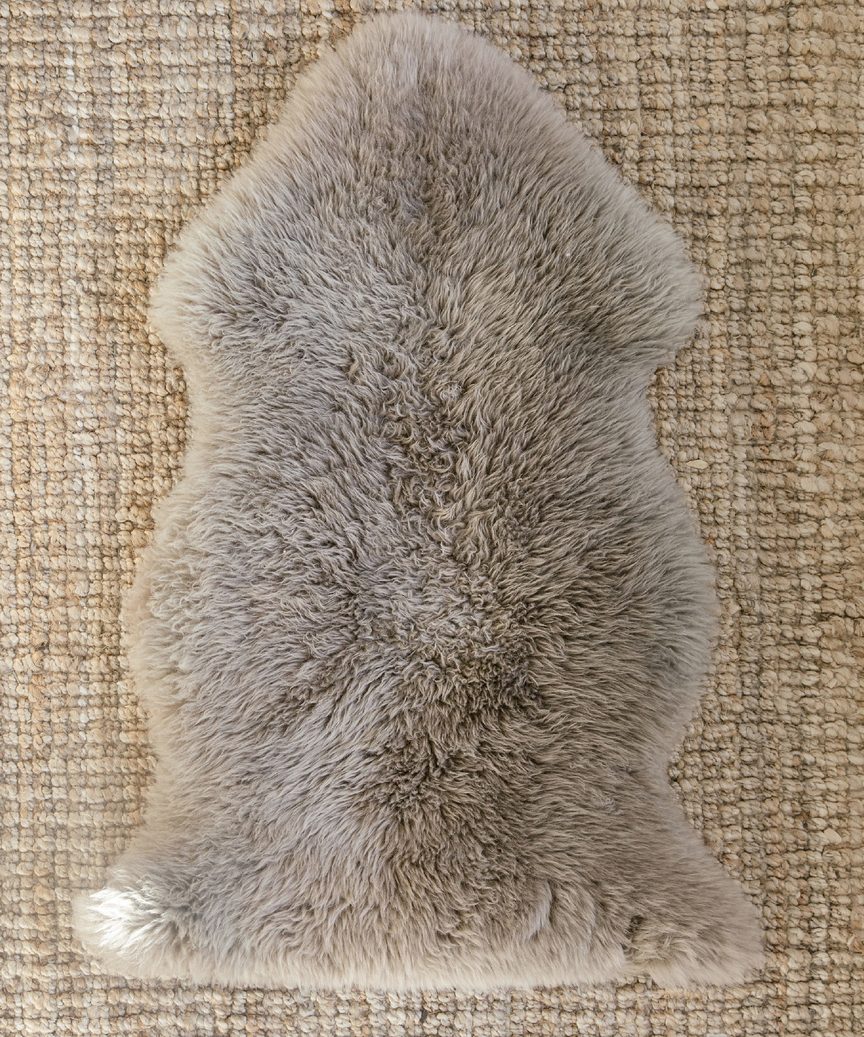The image depicts a downward view of a gray, furry material that closely resembles an animal fur or skin, possibly an animal tail or a thick, plush fabric. The piece is centrally placed on a beige and brown burlap-like fabric, creating a striking contrast. The shape of the fur is symmetrical along its longest dimension, aligning with the rectangular frame of the photograph. It forms a gentle pyramidal point at the top, curving inward and outward in a wavy, irregular fashion that gives it a somewhat phallic appearance or the silhouette of an upward-pointing arrow. This gray fur is adorned with subtle shades of light brown and white, adding depth and texture as light plays across its surface. The overall composition highlights the undulating, thick nature of the fur, accentuating its resemblance to an animal skin or a textured throw rug.